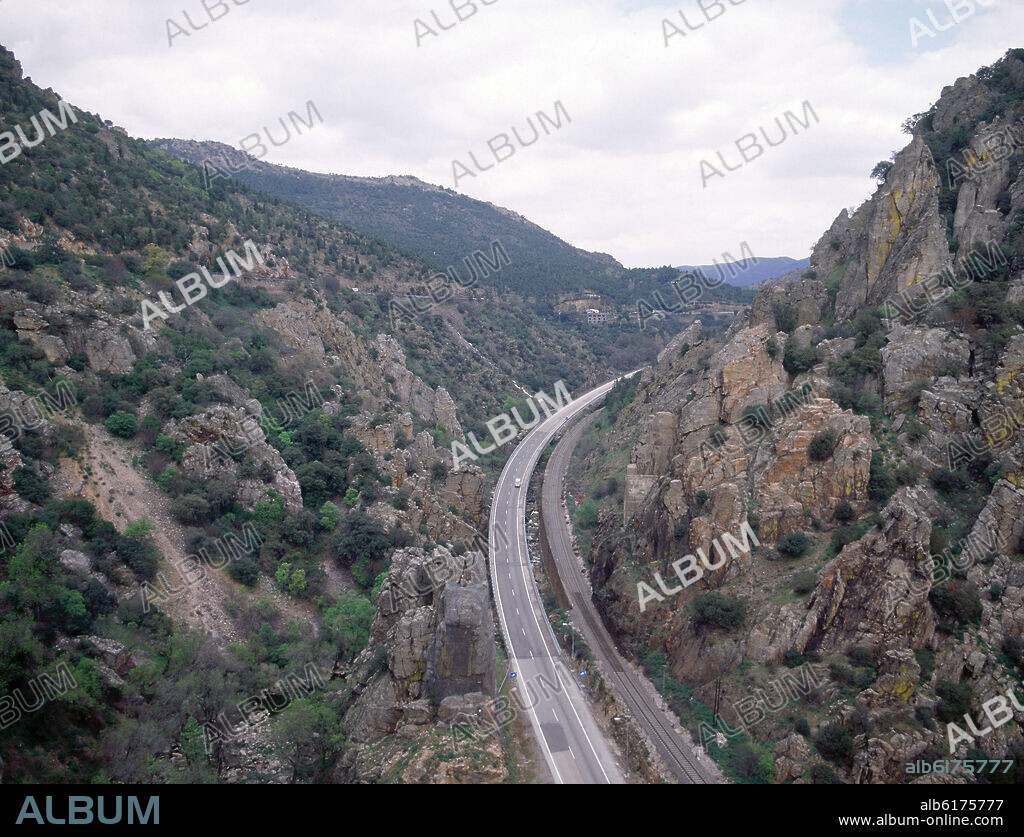The image presents an aerial view of a narrow gray highway cutting through a rugged mountain range, characterized by jagged, tan-colored rocks. The highway consists of two two-lane roads separated by trees and vegetation. One road heads north or toward the right corner, while the other leads southbound on the left. A small white car is visible on the highway, positioned around the middle of the photo, possibly struggling due to the narrow lanes. On the left side of the road, a ravine drops off several hundred feet, adding to the dramatic scenery. The terrain surrounding the highway is dotted with scattered trees and bushes, and the upper portion of the image features a skyline filled with dense, thick white clouds. The photograph is heavily watermarked with the word "ALBUM" in all capital letters, occasionally in teal, and appears semi-transparent in white and gray. Additionally, a small black box located at the bottom of the image contains an "ALBUM" logo on the lower left side and information about the photo and an album link on the lower right side. This meticulous watermarking serves to protect the photographer's work.